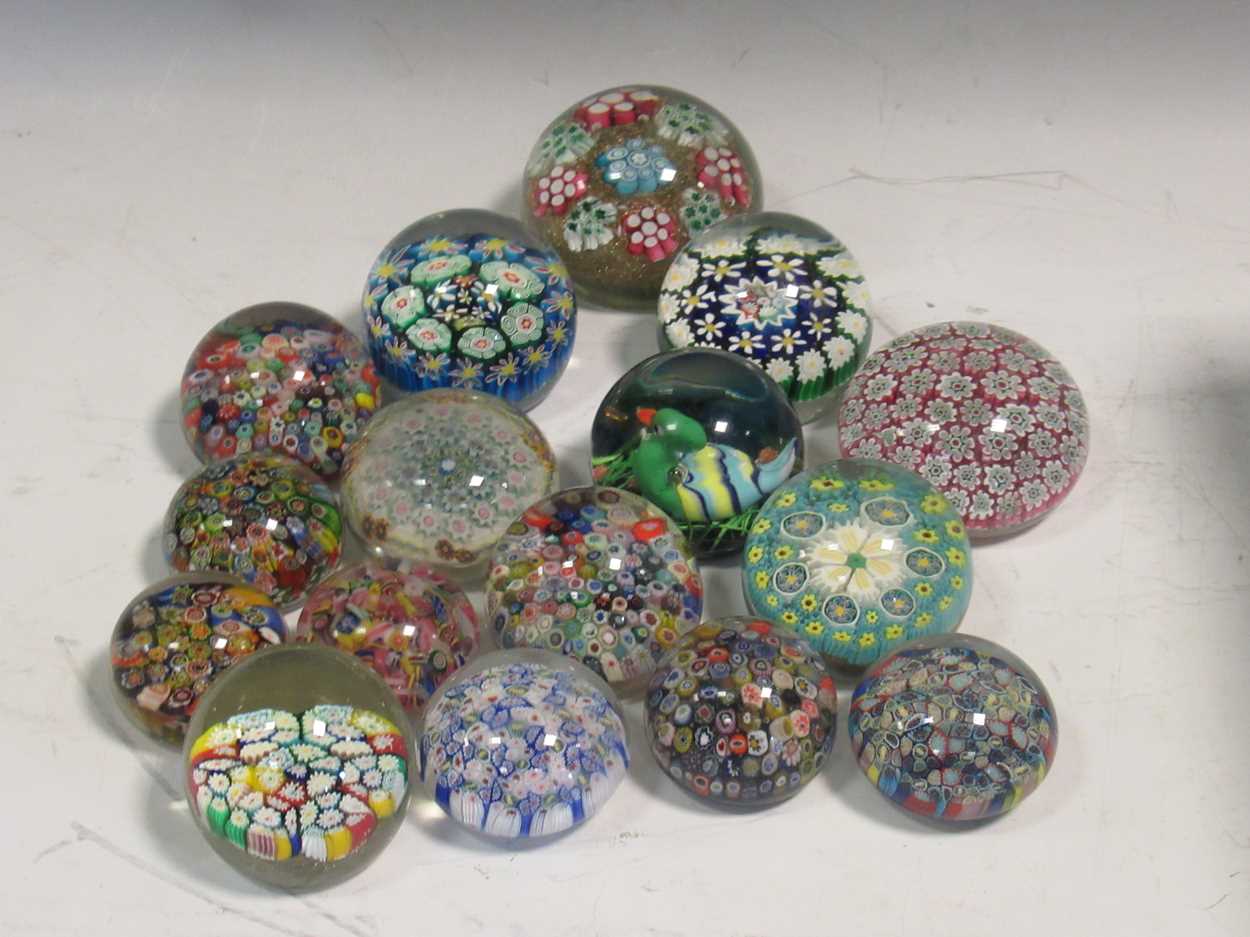A photograph captures an elegant collection of approximately a dozen glass paperweights, all featuring intricate designs encased within clear glass. These paperweights, varying in both size and shape—some spherical and others flattened at the bottom—are artfully arranged on a white table adorned with thin gray lines. Despite their differences, most of the paperweights display delicate floral designs using a type of resin to create the intricate scenes visible through the glass. Dominated by elegant bouquets, the designs include tiny white flowers, multicolored blossoms, and even specific patterns like pink flowers with white dots, blue flowers, and green ducks. One particularly striking piece features a dark blue base, encircled with white flowers that have green accents and a central white flower with a yellow dot. This exquisite collection, with its varied floral motifs and vivid color palettes such as teal with yellow flowers and magenta with white flowers, evokes a sense of timeless beauty and craftsmanship.